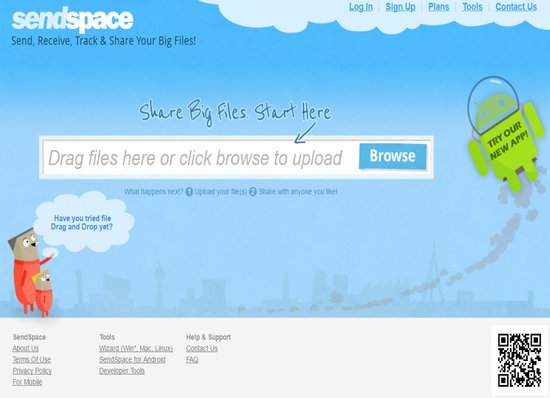This image displays the homepage of the website Sendspace. The header prominently features the service's functionalities, stating "Send, receive, track, and share your big files." To the right of the header, menu options include "Log In," "Sign Up," "Plans," "Tools," and "Contact Us."

Central to the page is a highlighted area prompting users to "Share big files, start here." This interactive section includes a data field where users can drag and drop files or click a blue "Browse" button to upload them. 

The website's background is a soothing light blue color. Beneath the central field, there's a step-by-step guide titled "What happens next?" illustrating the process: "1. Upload your files. 2. Share with anyone you like."

In the bottom left corner, an illustrated pair resembling a large and small person, both wearing orange onesies, ask "Have you tried file drag and drop yet?" through a speech bubble. On the right side, a green Android mascot wearing a space helmet is depicted launching upwards, with a caption encouraging users to "Try our new app."

The color palette of the site includes shades of blue, white, gray, orange, yellow, brown, and green. Elements of black are minimally present, if at all.